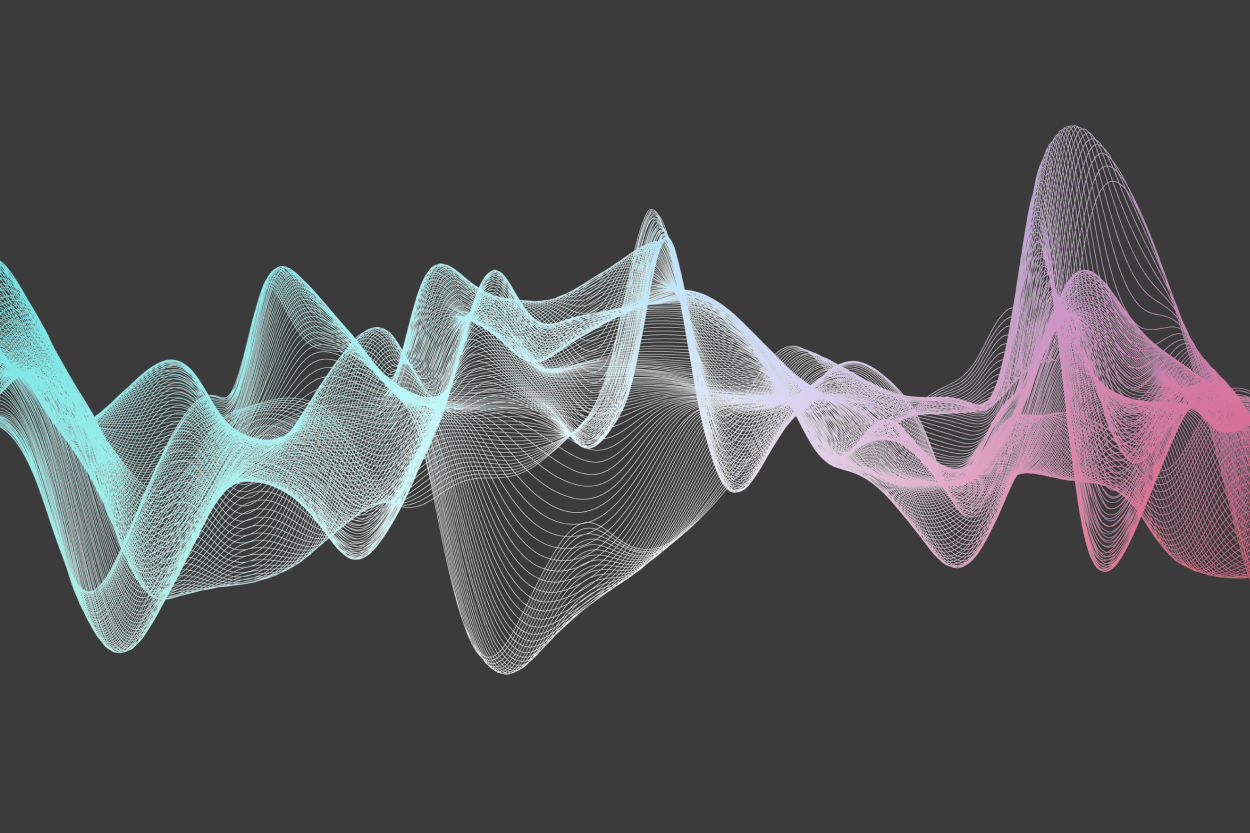This image depicts a 3D-generated visualization of waves, which could resemble sound waves or topographical contours, set against a dark gray background. The undulating, transparent waves flow gracefully from left to right, displaying varied heights and depths that create a sense of depth and dimension. On the left, the waves begin in a light turquoise or Tiffany blue hue, transition to white in the middle, and finally shift to pink on the right. The highest peaks are positioned in the pink section, while the lowest troughs occur in the white, though the turquoise region also dips significantly. The intricate lines within the waves suggest a motion akin to fabric billowing in the wind, enhancing the dynamic and fluid nature of the graphic.